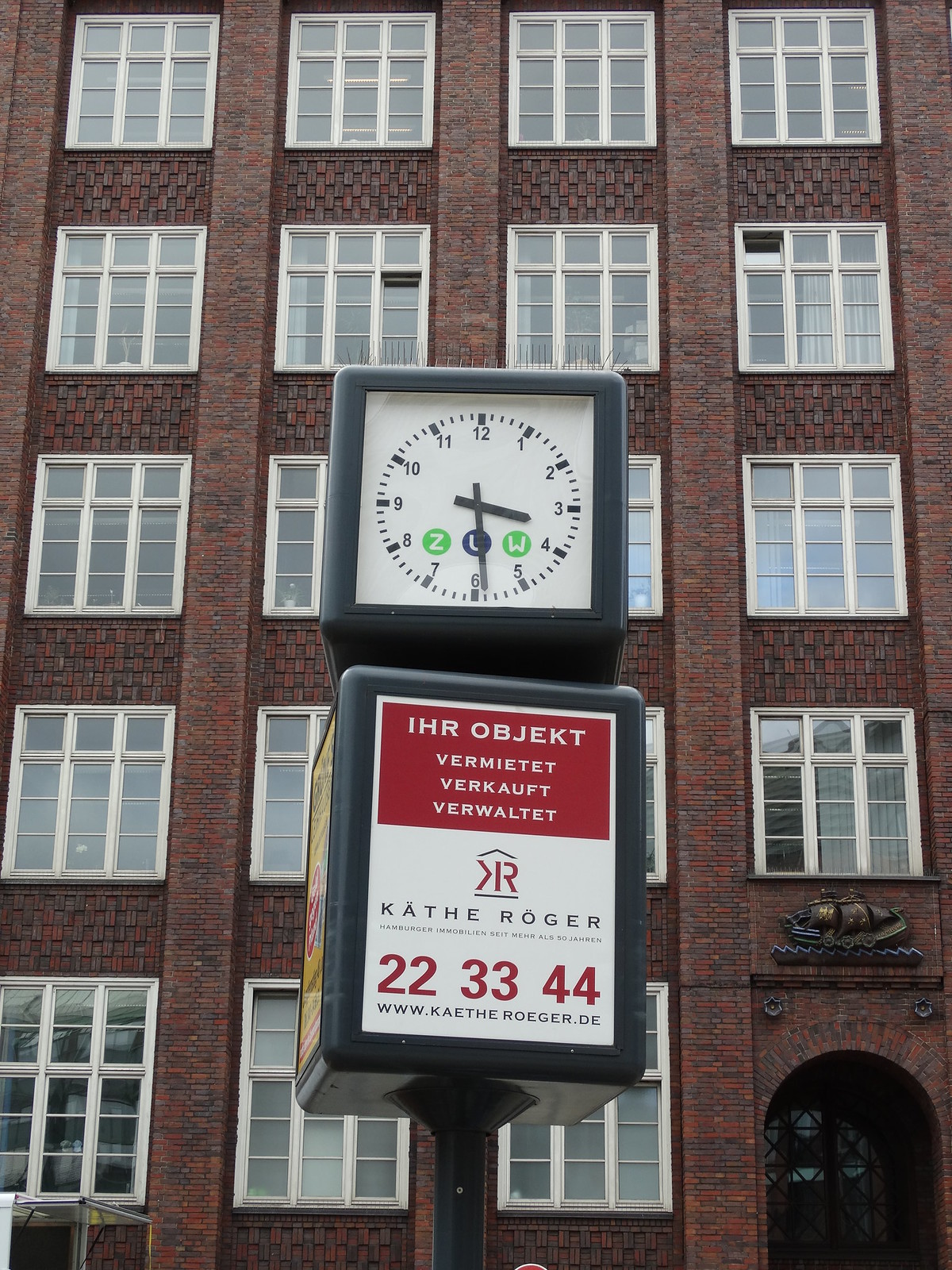In the foreground of the image stands a prominent clock post with a cube-shaped, white-faced clock displaying the time as 6:15. Below the clock, a rectangular extension of the post bears various advertisements in German, including the phrases "Z.U.W" and "Ihr Objekt," followed by "Vermietet, verkauft, verwaltet" and the contact information "22, 33, 44" as well as the website "www.kathereger.de." This structure features grayish trim and a gray body. Behind this post, a large, reddish-brown brick building with five visible stories rises into the frame, characterized by its many white, square-shaped windows, each potentially an individual apartment. In the bottom right corner of the photo, the building’s entrance can be seen, marked by an arched doorway with glass doors adorned with a black lattice pattern.